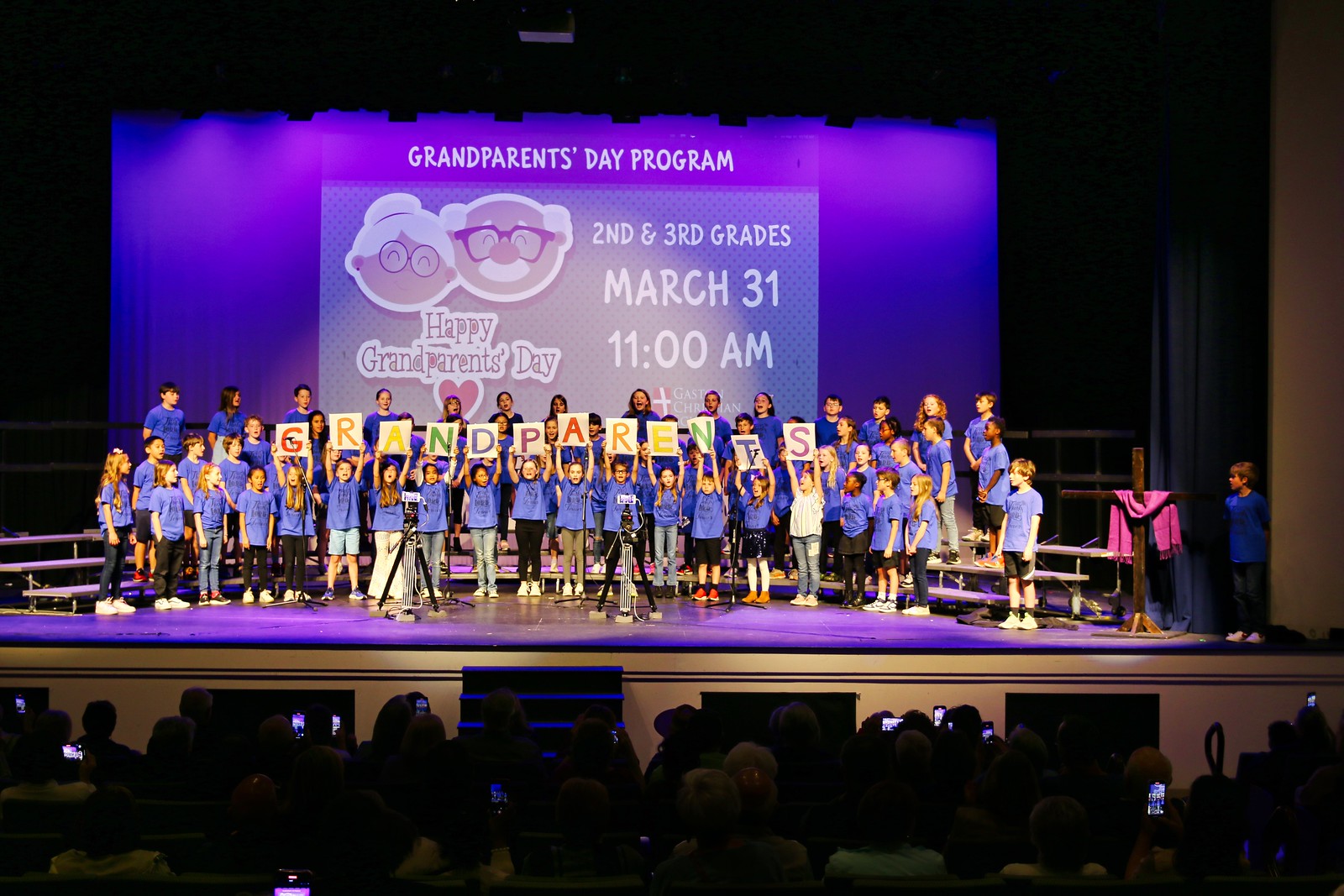The photograph captures an auditorium's vibrant Grandparents Day Program held on March 31st at 11 a.m., featuring second and third graders. The stage is adorned with purple lighting and a blue curtain, onto which the words "Grandparents Day Program" are projected in white font. At the center of the display are adorable cartoon figures of a smiling grandmother and grandfather, and below them, in red swirly font with a white border, the text "Happy Grandparents Day" appears. 

On the right side of the stage, in white font, the date and time—"March 31 11 a.m."—are marked, aligning with the presence of about 30 second and third graders on stage. These students, wearing blue shirts, are arranged in neat rows, and those in the front row hold up different colored signs that collectively spell out "grandparents" in rainbow letters. Positioned on the far edge of the stage is a notable cross with a pink ribbon draped over it. The audience, evidently engaged, captures the heartwarming scene with many holding their phones aloft to record the special moment.